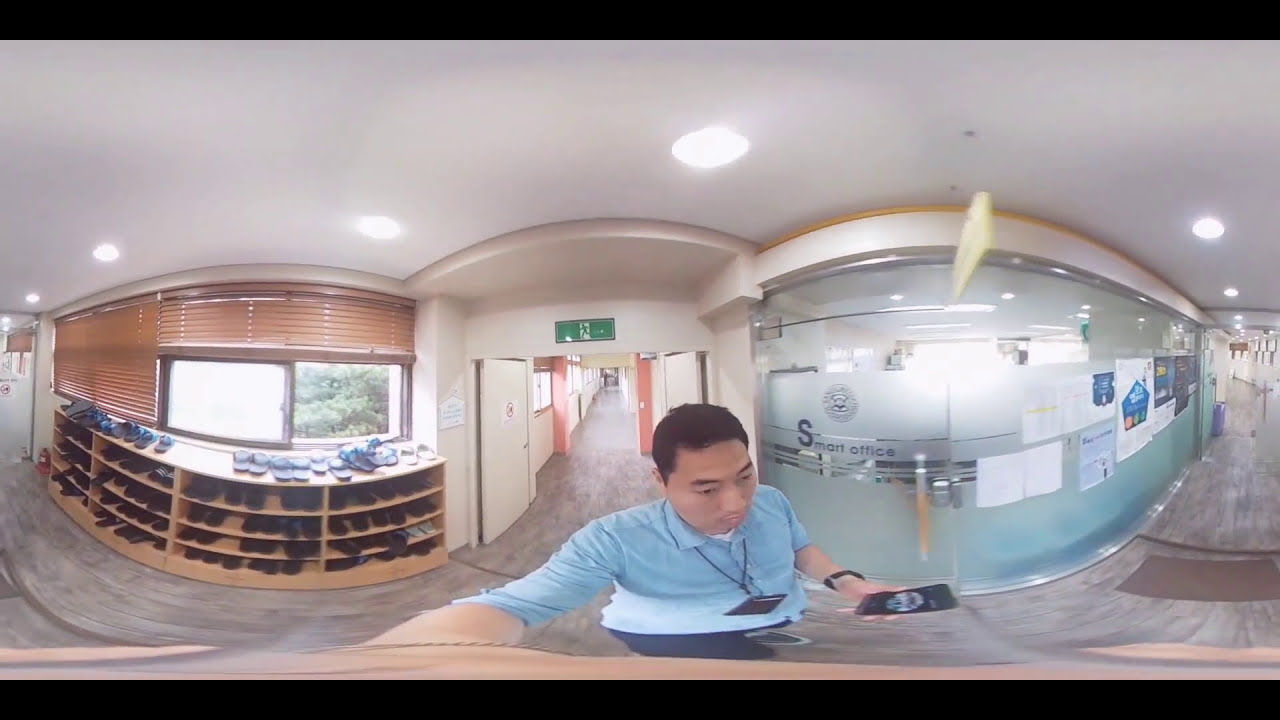The image depicts a young Asian man, estimated to be between 25 and 30 years old, walking through a modern office building. He is dressed in a blue shirt, wears a watch on his left wrist, and has a lanyard or badge around his neck. The office has a long corridor with beige walls, a white ceiling, and wooden floors. To his left is a distinctive glass wall that has "smart office" written on it and is cluttered with various papers; the glass is translucent at the bottom and transparent at the top. In his left hand, he holds his phone, and in his right hand, he holds a camera, which causes a noticeable warp effect in the image, particularly on his right arm and fingers. To the right of the man, there is a wooden rack filled with an assortment of shoes, including sandals and sneakers, likely placed there by office occupants. Behind him, the corridor stretches out, emphasizing the depth of the space and the structured layout of the office. The presence of windows on the right allows natural light to filter into the corridor.